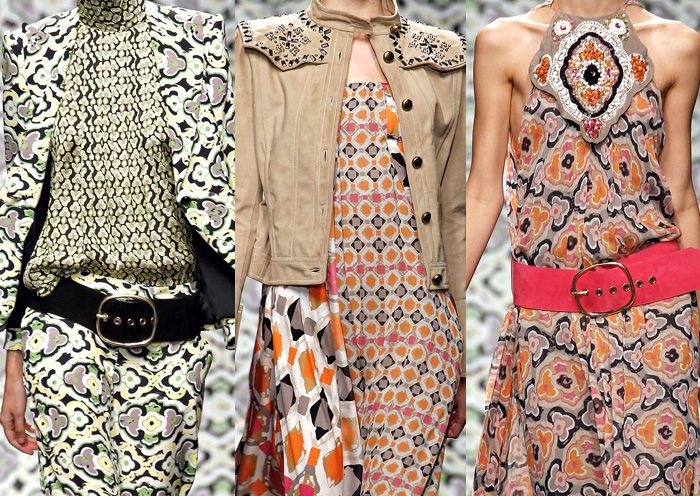This image portrays three models, possibly women, wearing various types of upscale clothing, showcasing intricate prints and a vibrant palette of colors. The models are positioned in a line, cropped at the neck and just above the knees, with their hands visible at the center of their bodies. The model on the left is dressed in matching pants and a jacket featuring a striking black and white snakeskin pattern, complemented by a large black belt with a texture that also suggests snakeskin. The middle model is adorned in a short tan leather jacket, paired with a skirt displaying a repeated floral pattern and an overlay that resembles a light shawl. The model on the right wears a sleeveless dress with an elaborate and colorful print consisting of orange, pink, tan, and black patterns. She sports a prominent, thick pink belt with multiple notches and a large medallion-like accessory around her neck. Each aspect of their attire—from the detailed patterns to the bold accessories—emphasizes the high-fashion style being modeled.